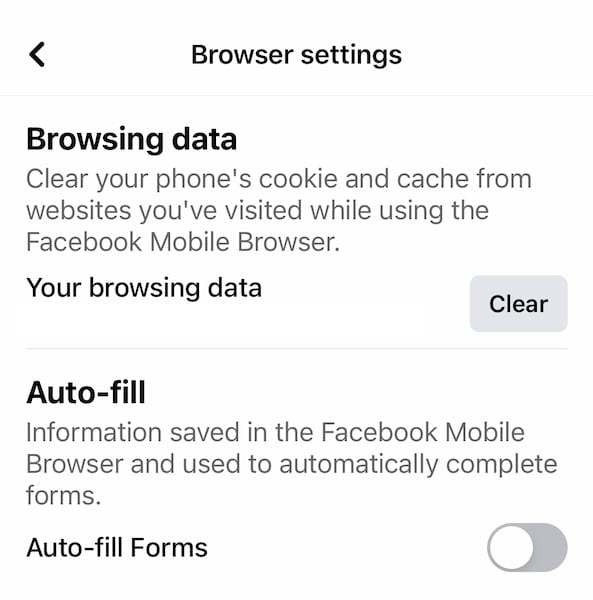Here is a detailed and cleaned-up caption for the described image:

"A screenshot of a smartphone or tablet screen displaying browser settings on a white background. At the top left, a back arrow indicates the option to return to the previous page. The center of the screen reads 'Browser Settings,' followed by the bold title 'Browsing Data.' Beneath this, in regular text, it states, 'Clearing your phone's cookies and cache from websites you visit.' The bold heading 'Your Browsing History' is below this text, and it is accompanied by a dark grey checkbox indicating that the option to clear browsing data is enabled. Further down, the section titled 'Autofill' explains that information saved in the Facebook mobile browser is used to automatically complete forms. However, unlike the 'Browsing History' option, the slider for 'Autofill Forms' is moved to the left, signaling that autofill is currently disabled.